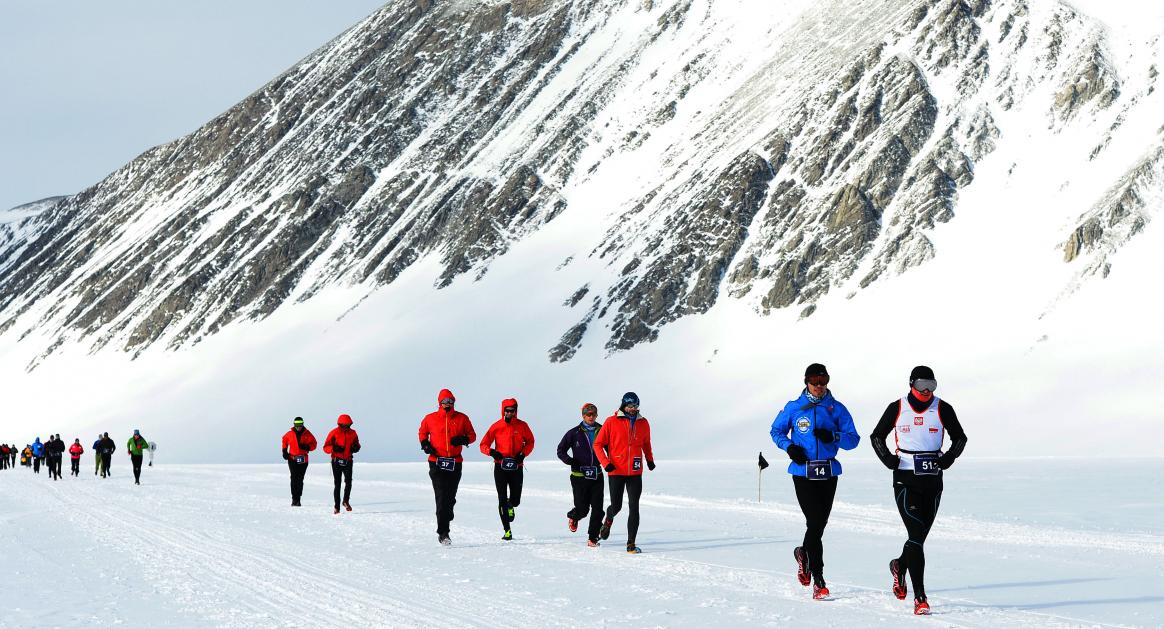In this photograph, a group of approximately 18 people is running on a wide, groomed snow-covered pathway at the base of a towering, snow-dressed mountain. The mountainside is rugged with visible rocky outcrops, and the sky above is a muted gray, hinting at overcast weather. The runners are dressed in a variety of ski outfits, primarily featuring red jackets with black pants, some with their hoods up. Near the front of the group, one participant wears a blue jacket with black pants, while another sports a white vest over black sleeves and black pants; both are notable for their red shoes. A tiny black flag is planted in the snow just behind the front runner with the blue jacket. In the background, slightly blurred figures add pops of green and blue to the scene, accentuating the line of participants making their way along the snowy trail. Scattered flags and the participants' visible numbered bibs indicate that this is likely an organized event, with everyone moving in the same direction.